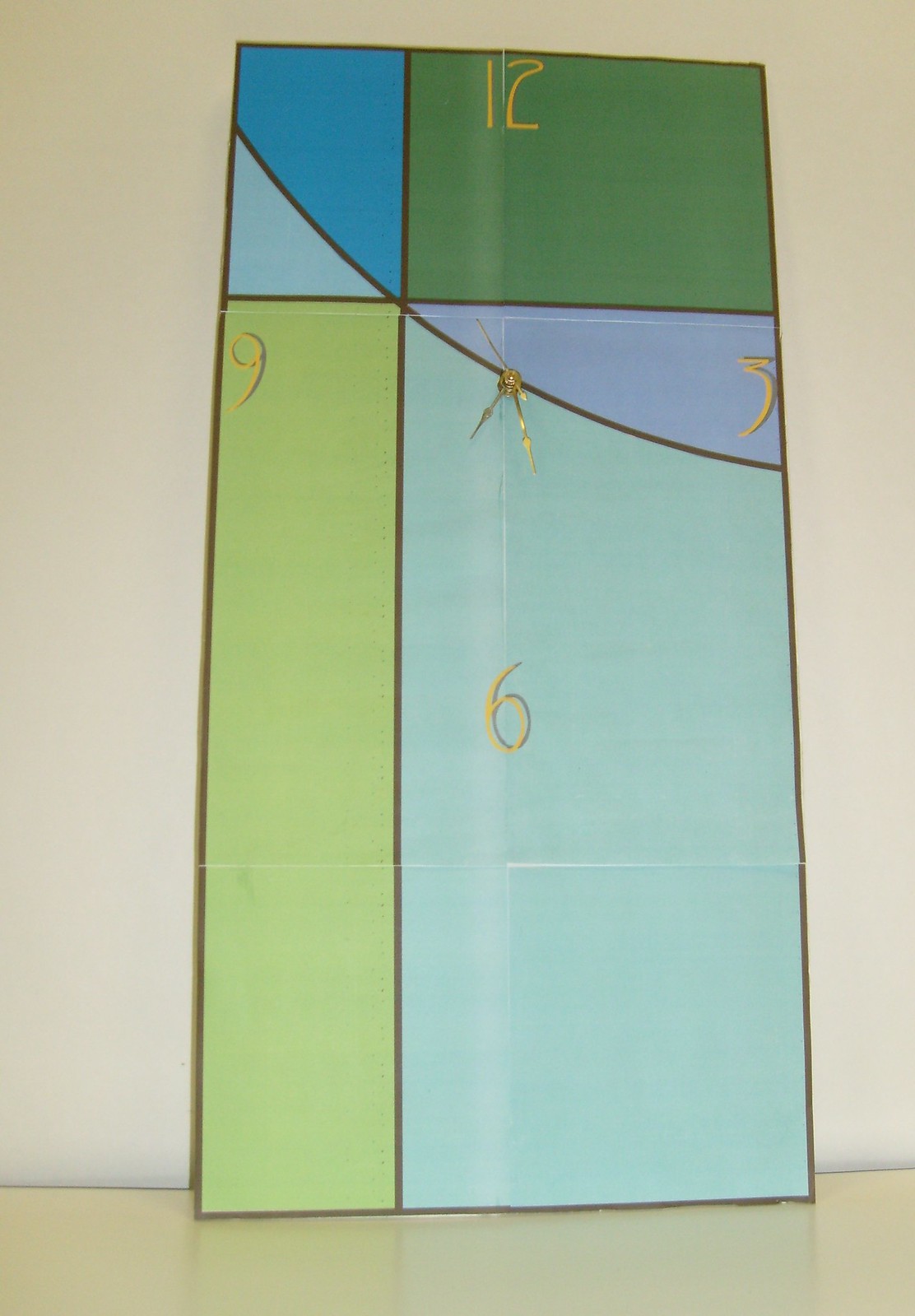The image showcases an exceptionally unique, rectangular clock that defies traditional designs. Unlike conventional circular clocks with numbers spaced evenly around the dial, this clock adopts a long, rectangular shape and bears a resemblance to a piece of stained glass. Its appearance is so unconventional that it might take a moment to recognize it as a clock. The clock face seems almost like a folded piece of paper, adding to its intricate design.

At the cardinal positions, the clock features the numbers 12 at the top (north), 3 on the right (east), 6 at the bottom (south), and 9 on the left (west). In the center, the clock retains the customary dial. The hands of the clock indicate the time is approximately 7:27. The background of the clock showcases an abstract, asymmetrical stained glass pattern with various shapes and swirls in a myriad of colors, contributing to its artistic and one-of-a-kind aesthetic.